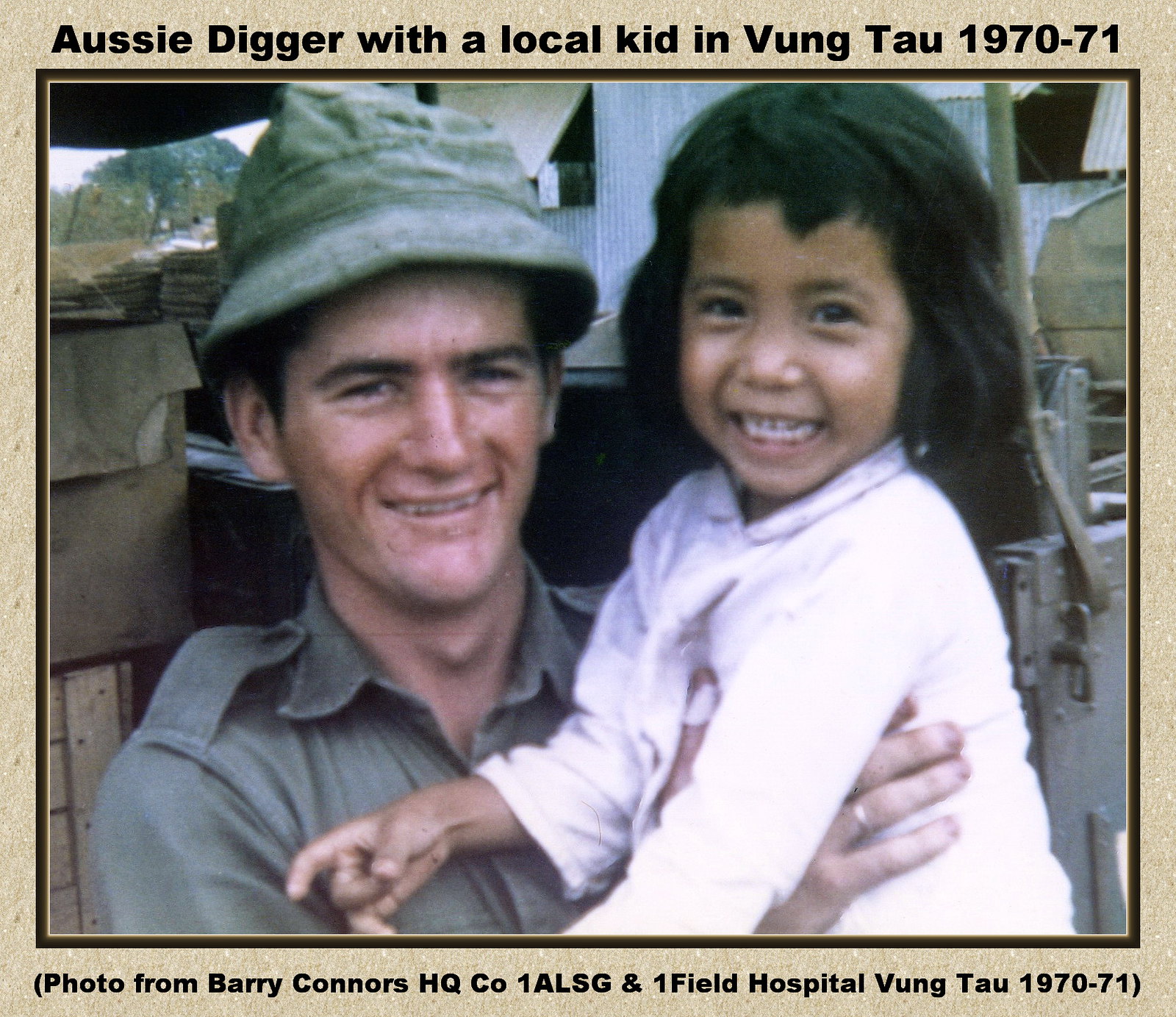This photograph, bordered in a light brown, textured frame, captures a touching moment in Vung Tau, Vietnam during 1970-71. The top of the image is labeled "Aussie Digger with the Local Kid in Vung Tau, 1970-71," while the bottom credits the photo to Barry Connors from HQ Company, 1ALSG, and 1 Field Hospital. The scene centers on a smiling Australian soldier, distinguishable by his green bucket hat and military uniform, holding a cheerful young Vietnamese girl. The girl, wearing a pink shirt and sporting dark brown hair, gazes happily at the camera. The backdrop includes military equipment and distant trees, indicating a barricaded area, and the photograph was taken during daylight hours. The camaraderie between the soldier and the child is palpable, set against the poignant backdrop of the Vietnam War.